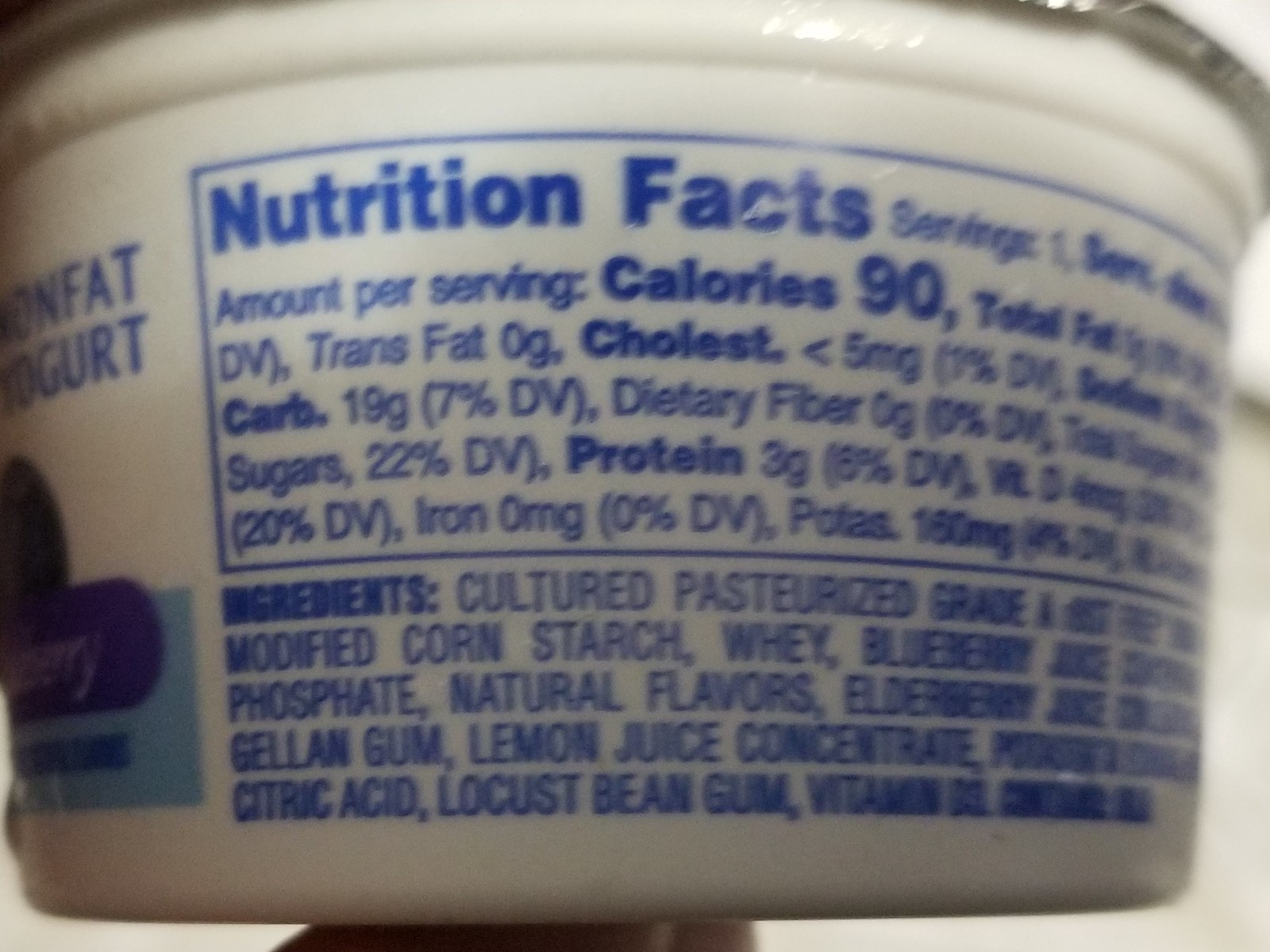This close-up color photograph captures the back of a small, white, single-serving tub of nonfat blueberry yogurt. The focus is on the nutrition facts panel and ingredients list, both of which are prominently displayed in blue text on the white plastic container. Although the image is somewhat blurry, some nutritional details are discernible, including that the yogurt contains 90 calories, 19 grams of carbohydrates, and 3 grams of protein. The ingredients list begins with cultured pasteurized grade A milk, modified cornstarch, whey, and blueberries, followed by lemon juice concentrate, natural flavors, citric acid, phosphate, and locust bean gum. To the left edge of the photo, the word "nonfat yogurt" is visible in blue, alongside a partially shown image of a blueberry and a purple panel that reads "blueberry" in white text. The background of the image is white, and at the bottom corner, a sliver of a person's hand can be seen holding the container up to the camera. A slight glimpse of the peel-off metal lid is visible at the top right corner.